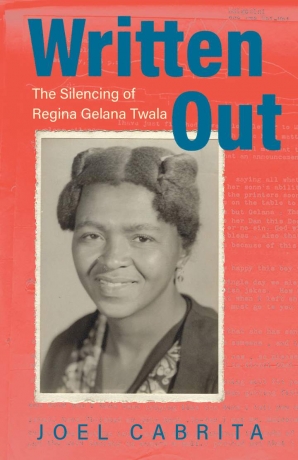This image is of a book cover with a tall, rectangular design and a faded red background. At the top, the book title "Written Out" is prominently displayed in blue text. Just below it, the subtitle "The Silencing of Regina Jelena Twala" appears in white. Central to the design is an old, black-and-white photograph bordered in white, depicting a woman, likely Regina Jelena Twala. She has dark hair styled in tight buns close to her head, with earrings adding a subtle adornment. Her high cheekbones reflect a touch of light, complementing her slight, pleasant smile that reveals her top teeth gently. Her attire features a brown jacket over a floral-patterned blouse. The background of the photograph is gray, lending a vintage feel to the image. At the bottom of the cover, the author's name, Joel Cabrita, is written in blue text. Faint white text is scattered across the red background, adding a final touch of detail to this compelling book cover.